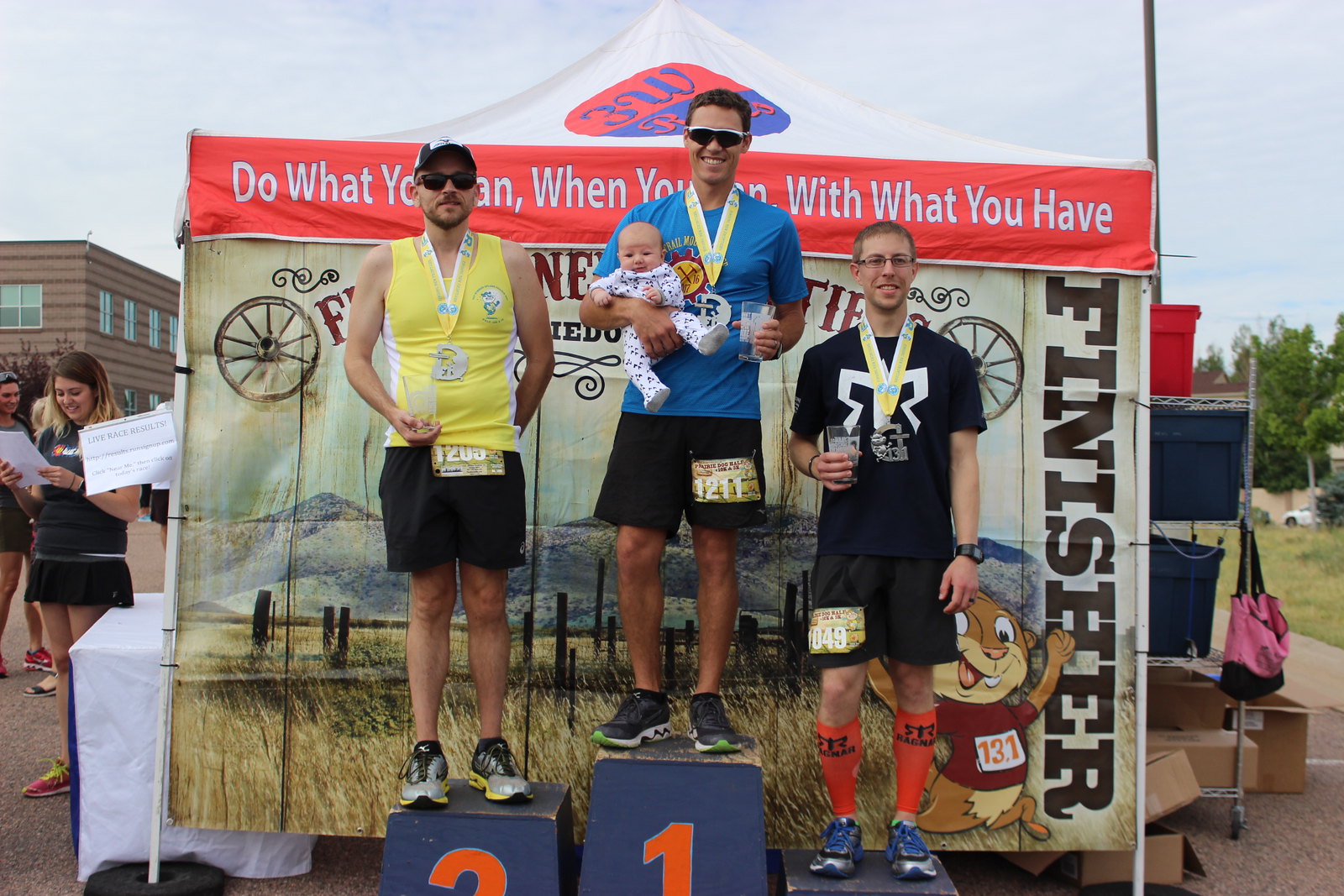Three men, positioned on a podium with labeled steps 1, 2, and 3, celebrate at the end of a race standing before a poster depicting an Old West background complete with cactus, wagon wheels, and prairie imagery. The vertical right side of the poster reads “FINISHER” in brown lettering, and a motivational quote, “Do what you can, when you can, with what you have,” is inscribed at the top. 

Each man wears black shorts. The first-place winner, on the highest step labeled “1,” is dressed in a bright blue t-shirt, holding a drink and a small baby. His race tag reads 1211. The second-place winner, on the step labeled “2,” sports black shorts, a yellow tank top, a hat, and sunglasses, and his tag reads 1205. Last, on the step labeled “3,” the third-place finisher wears black shorts, a black shirt with a reversed "R," and orange socks, and his tag reads 1049. All three men display their medals on yellow lanyards and hold beer glasses in their hands. A small cartoon chipmunk character is visible in the corner of the image.